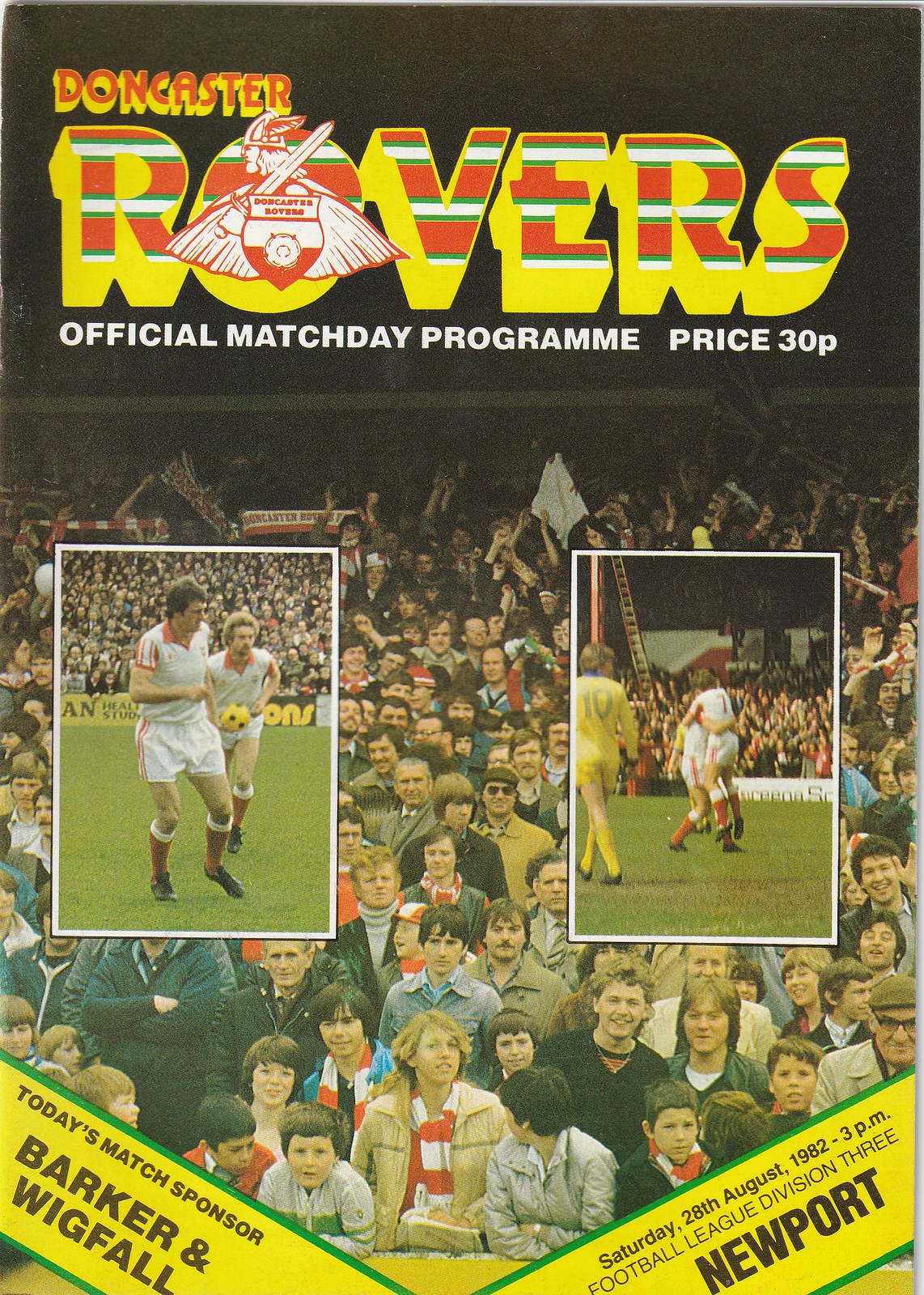The image is a cover for the Doncaster Rovers Official Match Day Program, priced at 30 pence. At the top, in bold red lettering with yellow shading creating a 3D effect, it says "Doncaster Rovers." The word "Rovers" is particularly striking, with additional green and white stripes and a Viking emblem featuring a sword and shield. Below the title, two smaller images with white borders are prominently displayed. The left image captures two soccer players in white uniforms with red stripes; one is holding a yellow soccer ball with black spots. The background is filled with a densely packed, excited crowd. The right image shows two players hugging, with another player in yellow walking to the left, set against a similarly enthusiastic crowd. The bottom two-thirds of the cover is dominated by a sea of spectators in the stadium, creating a vibrant and energetic atmosphere. A diagonal banner across the bottom states "Today's Match Sponsor: Barker and Wigfall" and includes the date of the Football League division match in Newport.